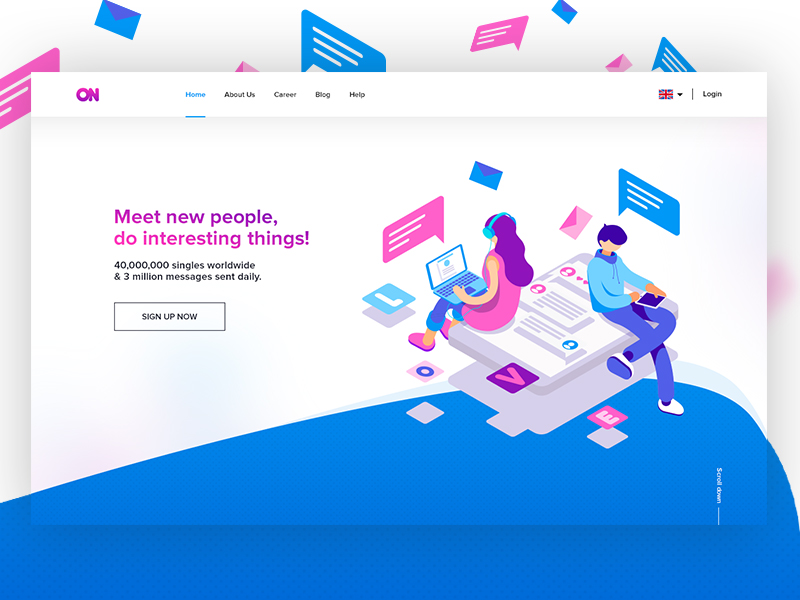The website features a predominantly white, pink, and blue color scheme. In the upper left-hand corner, the word "ON" appears in bold pink, all capital letters. To its right, "Home" is displayed in blue, followed by "About Us," "Career," "Blog," and "Help," all in black. The far right corner showcases a British flag with a small black drop-down arrow next to it, followed by a black slash and the option to "Log In."

The main page prominently displays an inviting message in bright pink lettering: "Meet new people, do interesting things!" Below this, it announces, "40 million singles worldwide, and 3 million messages sent daily." A call-to-action box encourages visitors to "Sign Up Now."

To the right of this text, there is an engaging illustration: two individuals sit back-to-back atop a large smartphone. The woman, adorned in a pink dress, with long purple hair and rolled-up jeans, is typing on a laptop while wearing blue headphones. She finishes her outfit with pink shoes. The man behind her sports a blue hoodie, blue jeans, and white sneakers, holding an iPad with his leg crossed over the other. He has bluish hair, and both characters' feet rest on a blue floor. Scattered on the floor are a pink letter "E" and a blue letter "O," adding a playful element to the scene.